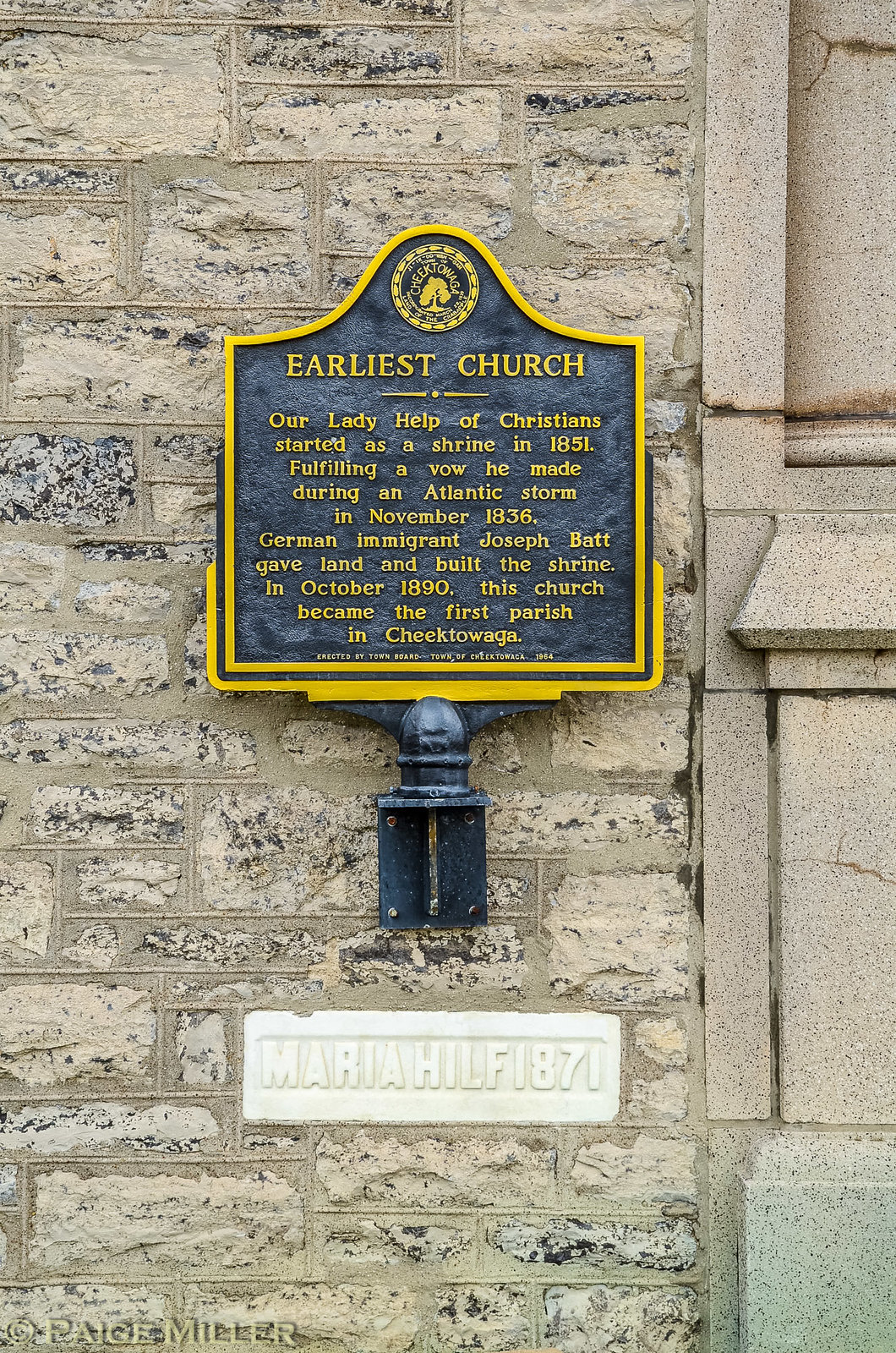On the side of this gray brick building, there's a detailed plaque with a distinctive gold border and a deep blue center. At the top of the plaque is a crest that reads "Cheektonga," spelled C-H-E-E-K-C-O-W-A-G-A. Beneath the crest, in yellow text, are the words "Earliest Church." The inscription tells a historic story: "Our Lady's Help of Christians started as a shrine in 1851, fulfilling a vow made during an Atlantic storm in November 1836. German immigrant Joseph Batt donated the land and constructed the shrine. In October 1890, this church became the first parish in Cheektonga." Just below this main text, it reads "Maria Hilf, 1871." The plaque is an iron board shaped with an arched top, enhancing its historic and decorative appeal, with the text also showing in bright yellow.